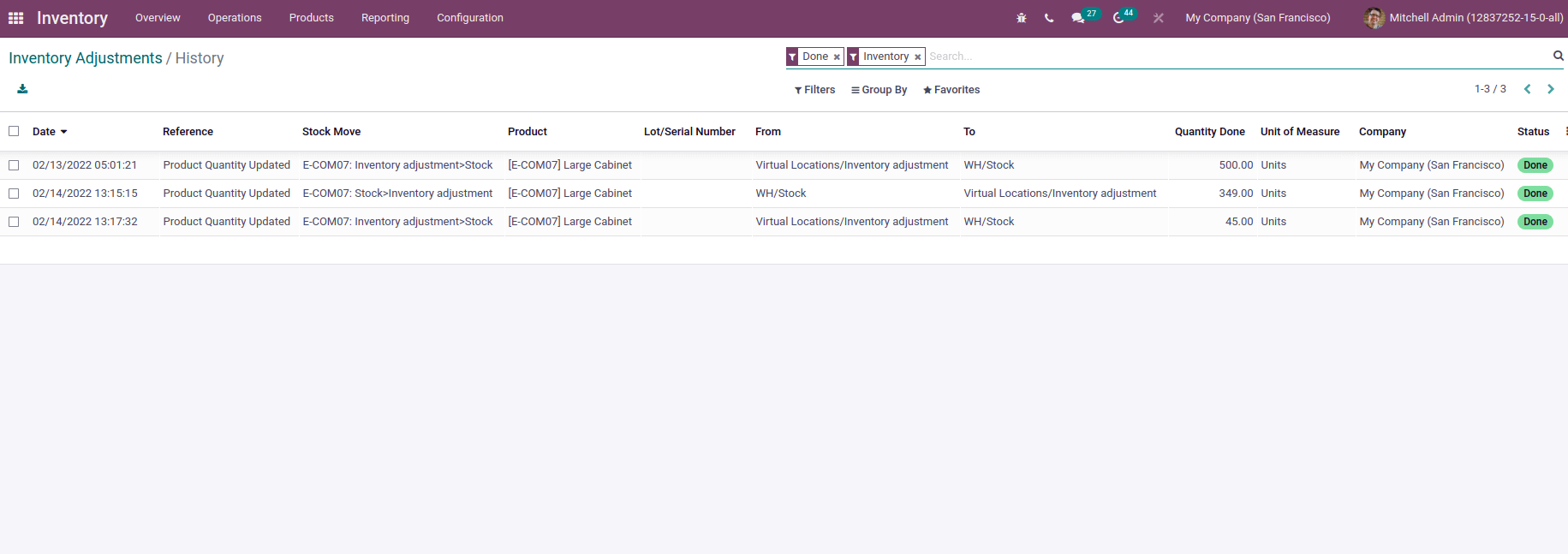This image is a detailed screenshot of a web page, displaying the dashboard interface of an inventory management system. The top header is a prominent purple bar. On the left side of the header, written in white, are the words "Inventory." The navigation menu within the header includes tabs labeled from left to right as "Overview," "Operations," "Products," "Reporting," and "Configuration."

On the far right side of the header, the user's account name is displayed, although the last name is difficult to read due to its small font size, but it seems to start with "Mitchell."

The main background of the web page is white. Just below the header, on the left side, written in blue font, is the text "Inventory Adjustments / History." Below this title, a spreadsheet-like table is present. This table includes three rows and several columns. The columns are labeled from left to right as follows: "Date," "Reference," "Stock Move," "Product," "Lot / Serial Number," "From," "To," "Quantity Done," "Unit of Measure," "Company," and "Status."